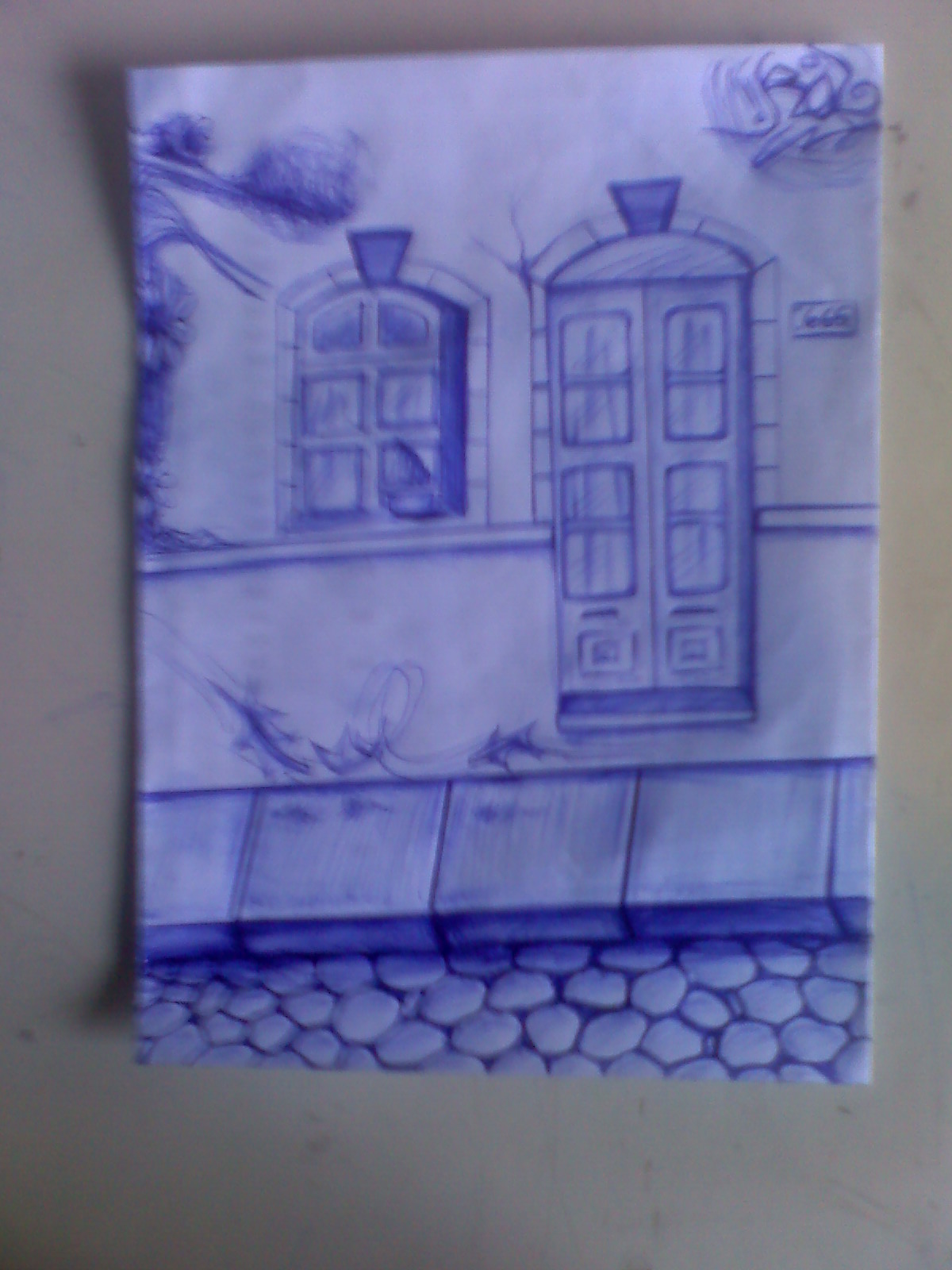A detailed ink drawing on a folded napkin sits atop a white table, slightly curled at the corners. The drawing depicts a scene featuring a cobblestone road formed by ovals and circles at the bottom. Adjacent to the road is a sidewalk delineated by four and a half concrete squares. Above the sidewalk, scribbles hint at graffiti or smoke, adding a chaotic touch. A building stands prominently, characterized by a rectangular door with an arched top, encased in bricks. The door features eight small window panes arranged in pairs, suggesting intricate design details with slight hash marks framing it. Next to the door on the left is a similarly arched window with six panes, capped by a shaded downward-pointing triangle. The building scene continues to the left, showcasing a tree with visible foliage and a small flower. The entire sketch is rendered in blue ink, with the napkin producing subtle shadows on the white table.